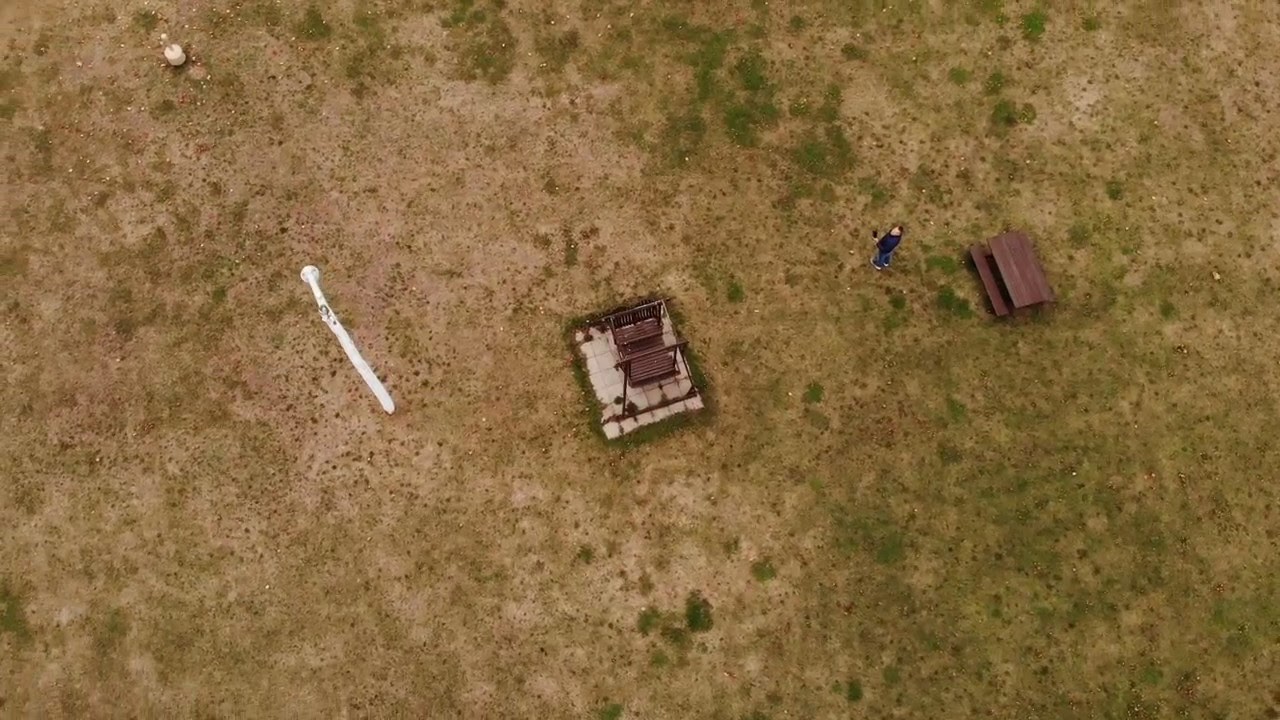The image presents a bird's eye view of an outdoor setting characterized by a mostly dry, patchy grassed area interspersed with occasional green patches. Central to the image, there is a paved area composed of white square blocks, which houses wooden furniture, likely seating. To the right of this paved section stands a person, who appears to be male, dressed in dark clothing consisting of a dark top and jeans. This individual seems to be gazing up at the camera, possibly indicating the use of a drone. Adjacent to him is a brown picnic bench. On the left side of the paved area, there's a white pole or post whose purpose is unclear. Additionally, near the top left corner, there's another unidentified white object with a long handle.